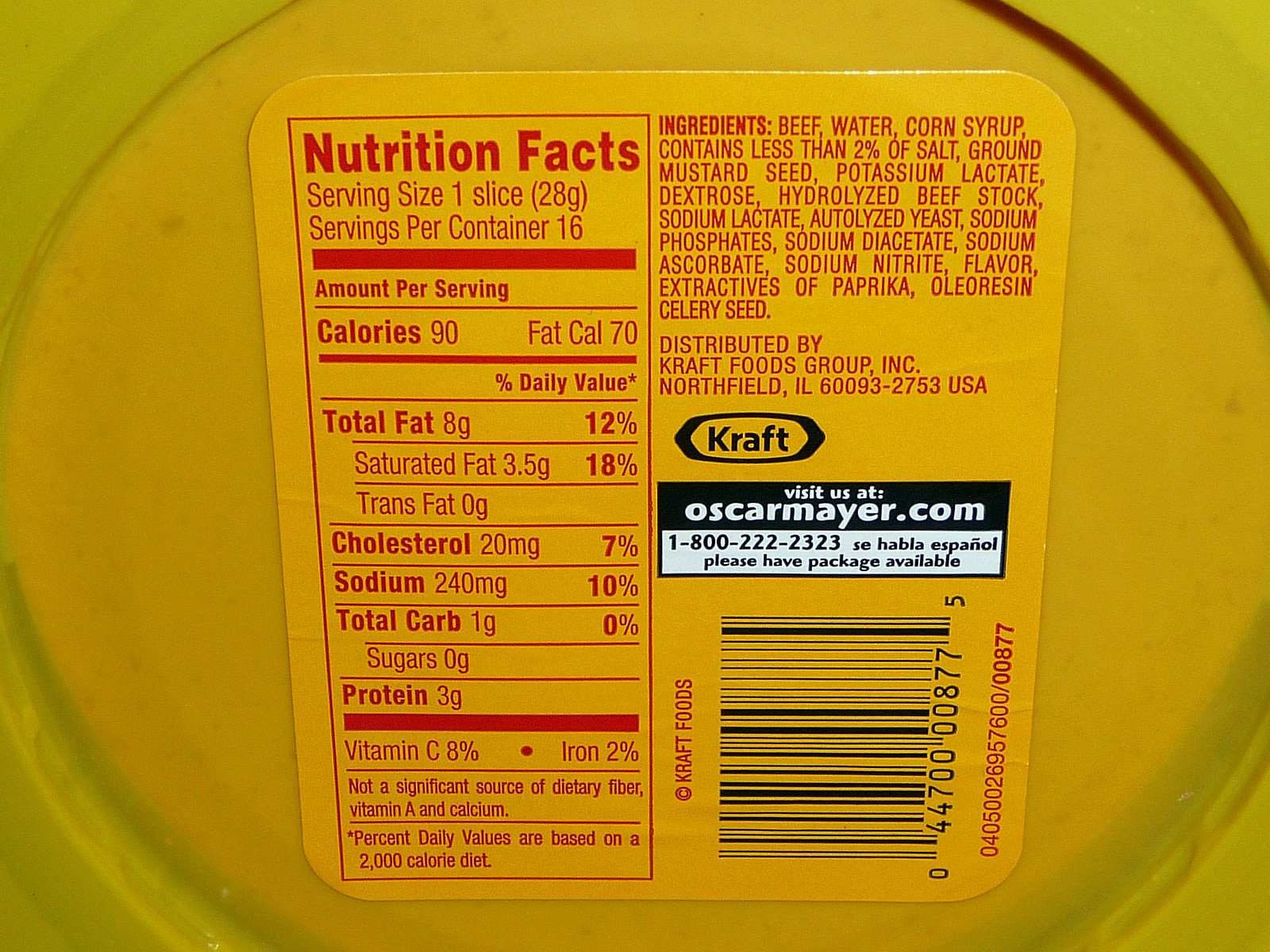This image features the rear view of a package likely produced by Oscar Mayer. The packaging is prominently yellow with red print, suggestive of a bologna product, although it is not explicitly labeled as such. The shape of the package is notably round, typical of sliced meat packaging. Nutritional information is visible, indicating high sodium content and calorie details for one slice, reinforcing the assumption of it being bologna. On the right side, an ingredient list reveals components such as beef, water, and corn syrup. Additionally, the package provides a contact address for Kraft Foods in Illinois and displays a black Kraft logo. There are also instructions for customers to visit oscarmayer.com or to call a toll-free number for product inquiries.